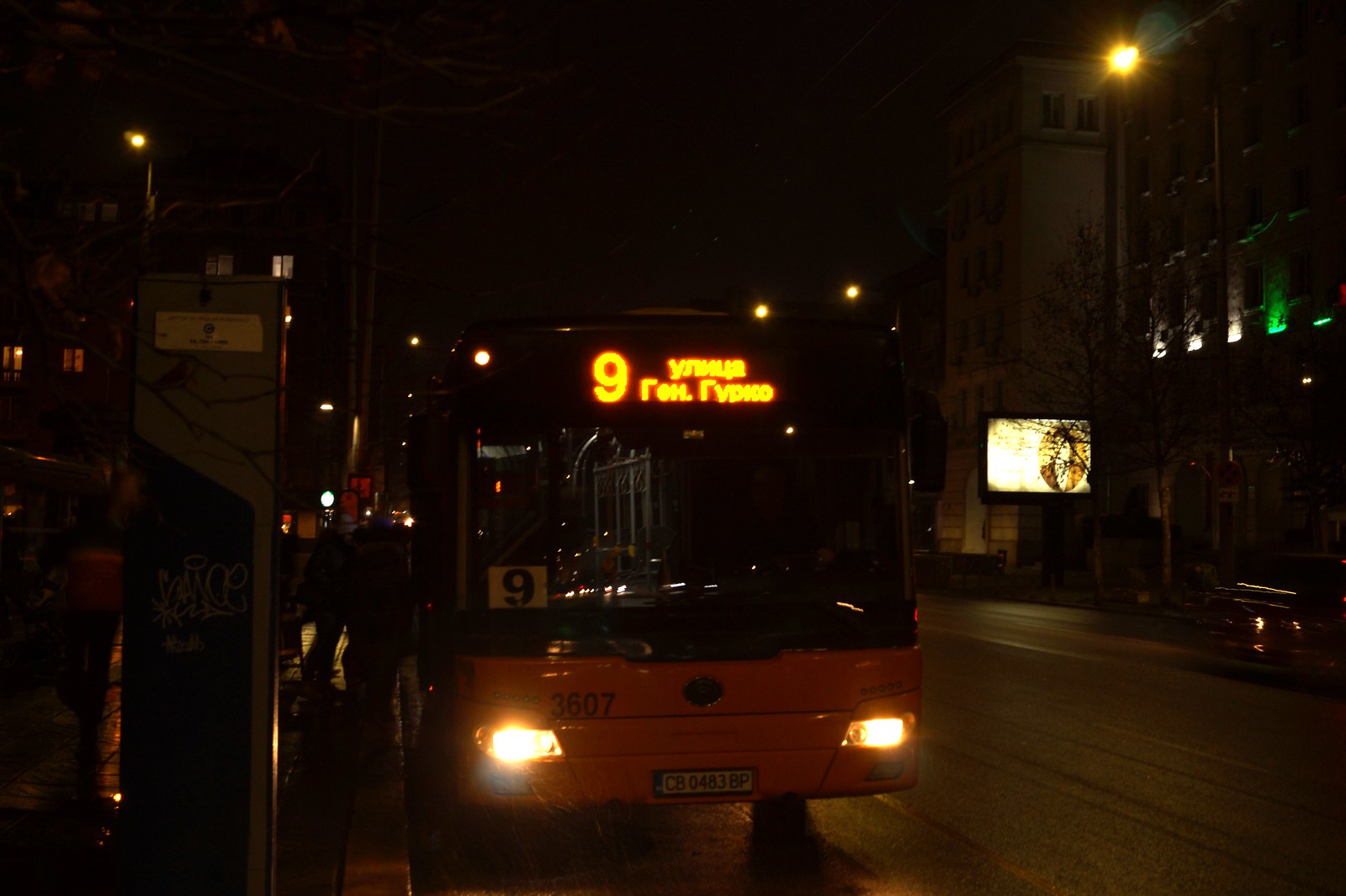This nighttime urban photograph captures a dimly lit city street, predominantly displaying the front of a municipal yellow bus with the license plate CB0483BP and the fleet number 3607 marked on its lower white bumper. The bus, possibly either in motion or stationary, prominently features a digital display at the top indicating the route number "9" followed by words in an unidentified foreign language. The brightly shining headlights illuminate the surrounding dark street, which is paved with black asphalt. To the left of the bus, a faint silhouette of the driver is visible, though there appear to be no passengers. Several people are seen standing and walking on the sidewalk alongside a graphitized metal structure, possibly an old phone booth or electrical equipment. Emerging behind these figures is an apartment building with a few lit windows. The right side of the street reveals another building adorned with a lighted billboard showing the head and bust of a human figure within an oval frame. A potential blur of a passing car adds subtle dynamism to this otherwise still scene, enhanced by several streetlights and various signs illuminating the dark ambiance of the city night.